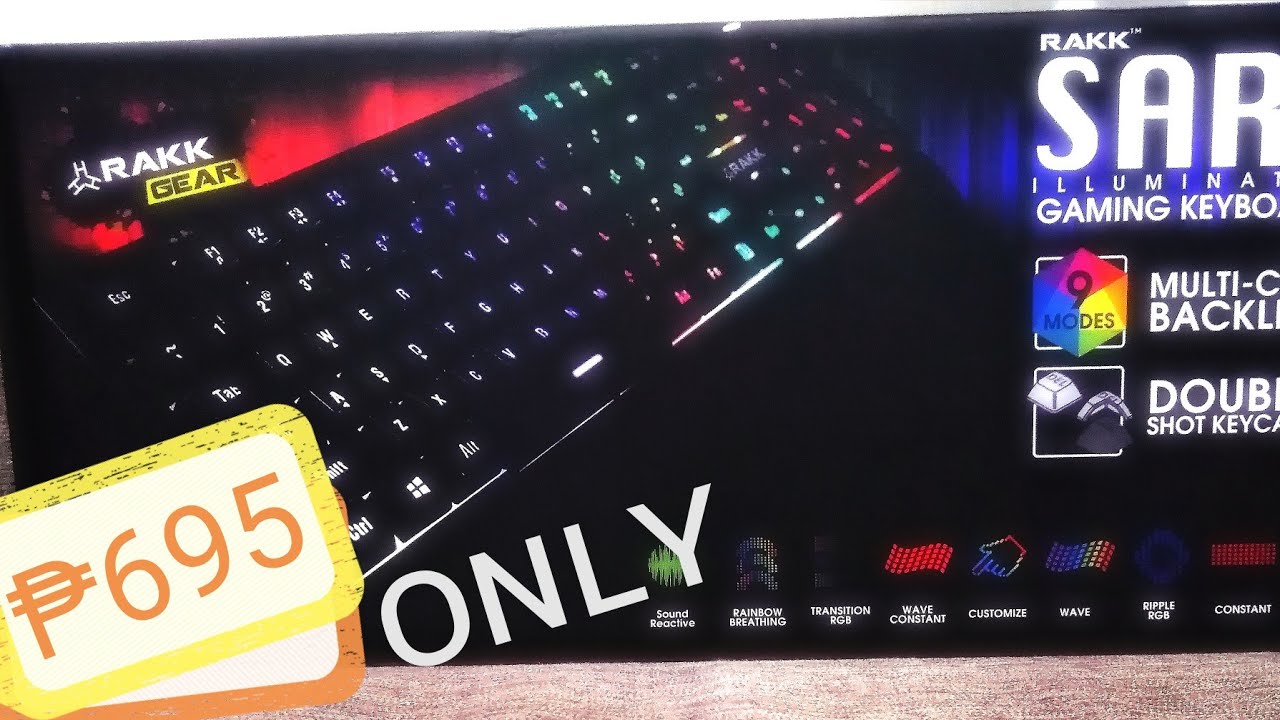In the image above, the background is completely black, creating a stark contrast with the elements in the foreground. On the left side, positioned diagonally, is a standard keyboard featuring keys with various colors. It is unclear if these keys are illuminated or simply multi-colored. Behind the keyboard, red clouds with a fiery appearance add a dramatic effect, enveloping the logo of the brand "RAKK."

Additionally, in the bottom left-hand corner, there is a yellowed border resembling a price tag, stating "$6.95 only," with a stylized "P" that has two lines through it. On the right side of the image, the text "RAK SAR illuminated gaming keyboard" confirms that the keyboard is indeed backlit with multiple colors. Further text indicating "double shot key" is partially visible, though the remaining words are obscured.